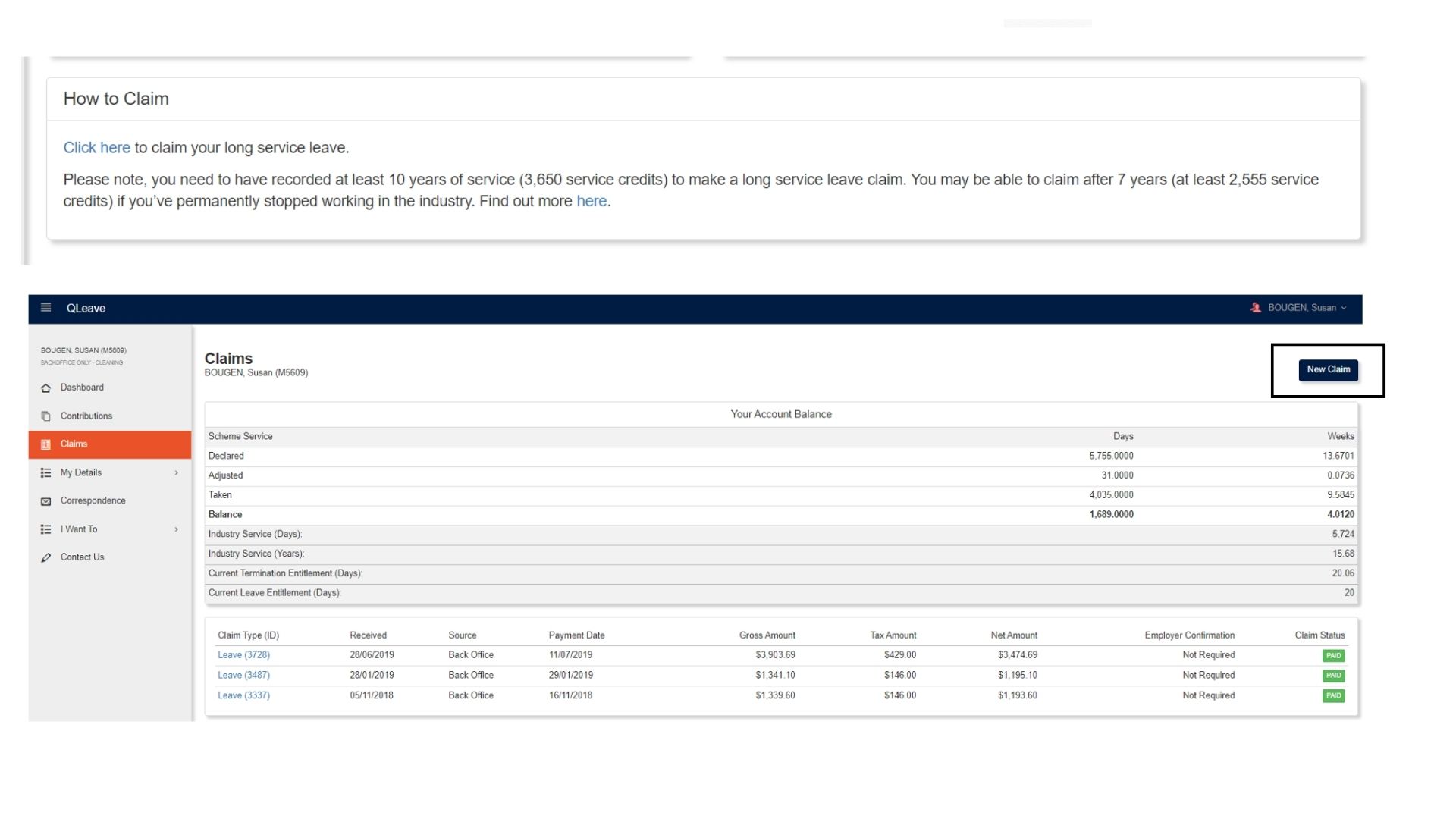**Detailed Caption for the Claims Website Screenshot:**

The image portrays a computer screen displaying a webpage dedicated to long service leave claims. The background is predominantly white, with a main section at the top center containing a thin gray-outlined white box. Within this box, the title "How to Claim" is prominently displayed in bold black letters at the top left. Directly below, the text "Click Here" appears in blue, followed by "To Claim Your Long Service Leave" in gray. Another gray text line reads, "Please note, you need to have recorded at least 10 years of service (3,650 service credits) to make a long service leave claim. You may be able to claim after seven years (at least 2,555 service credits). If you've permanently stopped working in the industry, find out more here," with "here" highlighted in blue to indicate a hyperlink.

Beneath this section, another panel is visible, topped by a dark blue bar spanning its width. The left side of this bar features a white icon with four horizontal bars, accompanied by the label "Cue Leave" in white letters. On the right side of the bar, a small pink person icon appears next to the capitalized name "BOUGEN," followed by "Susan" and a down arrow, indicating a dropdown menu for the user Susan Bougen.

The area directly below this blue bar is divided into two sections. On the left is a light gray vertical panel displaying user-specific information: "Susan Bougen," "Identifier M-5609," and "Back Office Only Cleaning." This panel includes navigation options such as Dashboard, Contributions, Claims (highlighted in orange), My Details, Correspondence, I Want To, and Contact Us, with Claims highlighted to denote the current selection.

The right section features a large, landscape-oriented display entitled "Claims" for "Bougen Susan, M-5609." In the far-right corner, a dark blue box contains a button labeled "New Claim" in white text. Below this, several lines detail account information, starting with a section for "Your Account Balance" on a white background. Further down, a gray background row lists column headings: "Scheme," "Service," "Days," and "Weeks." The subsequent rows on a white background feature data under labels "Declared," "Adjusted," "Taken," and "Balance," with corresponding days and weeks.

Following this, another light gray panel provides additional details under headers such as "Industry Service Days," "Industry Service Years," "Current Termination Entitlement Days," and "Current Leave Entitlement Days," each with relevant numbers of weeks in the last column.

Finally, a detailed table appears with several columns labeled "Claim Type," "Received," "Payment Date," "Gross Amount," "Tax Amount," "Net Amount," "Employer Confirmation," and "Claim Status." This table enumerates three claims dated 06-28-2019, 01-28-2019, and 11-05-2018, each noting the financial details and displaying a green box with the word "Paid" in the Claim Status column, indicating that all listed claims have been settled.